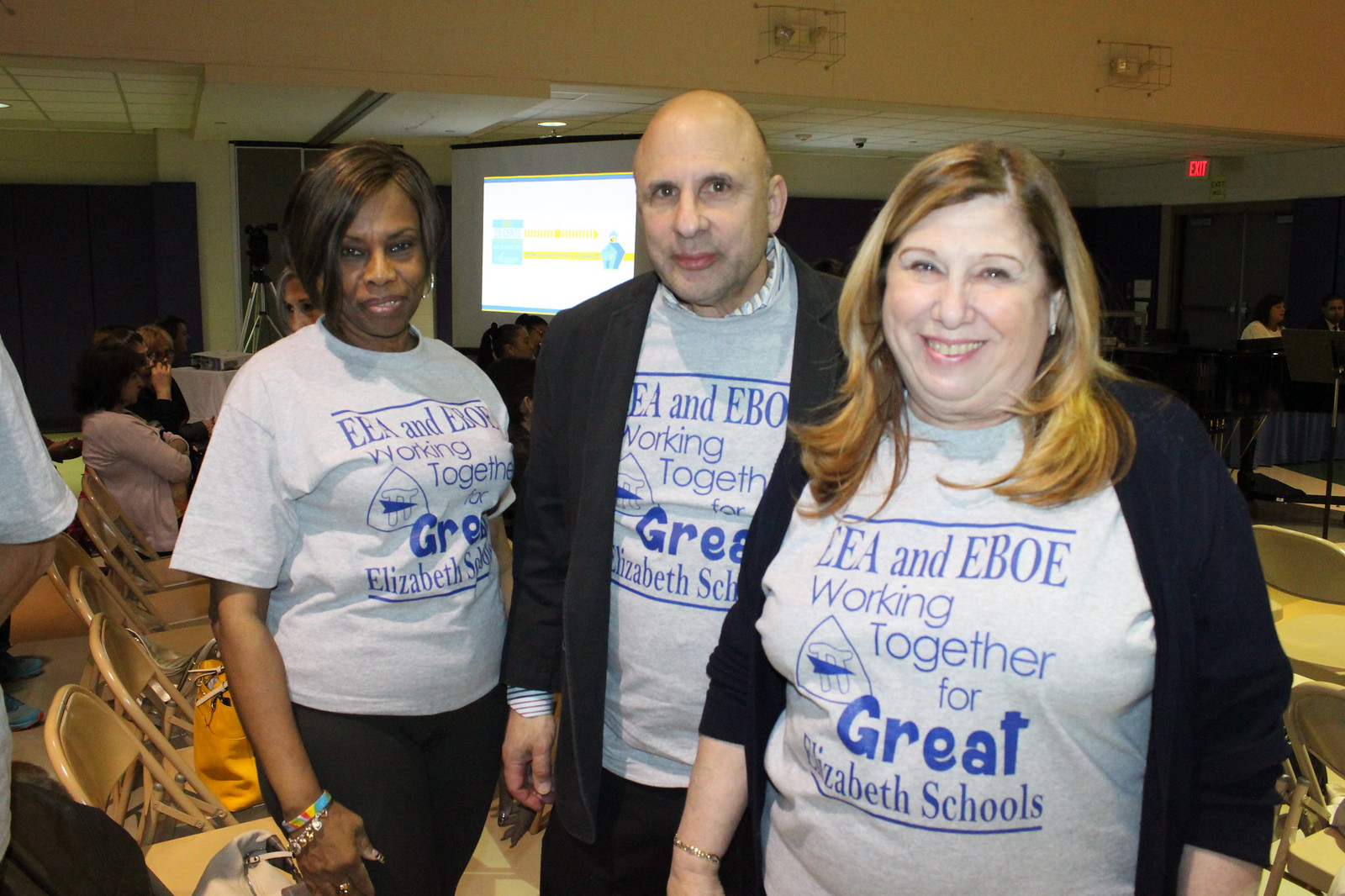In this photograph, three adults stand side by side, likely during a meeting or conference related to the Elizabeth Schools. They are all wearing light gray t-shirts emblazoned with the message "EEA and EBOE Working Together for Great Elizabeth Schools." The lettering on their shirts features a darker blue for the word "great," making it stand out. Each shirt also displays a triangle emblem with a blue arrow through it and possibly a Jewish or Greek symbol, although the details are not entirely clear.

The group consists of a bald Caucasian man in his late 40s to mid-50s standing in the center, flanked by two women. To his left is a white woman in her 40s with blonde, shoulder-length hair, who wears a blue sweater over her t-shirt. On his right is an African woman with dark hair parted on the side, dressed in black leggings, accessorized with two bracelets—one multicolored and one beaded.

The background reveals a low-ceilinged, dimly lit room filled with metal beige folding chairs, some of which are occupied. A yellow bag is casually left on one chair. Behind the group, a stage is visible where a woman appears to be standing near a piano, possibly preparing for a presentation. A screen or projector further suggests that a presentation or assembly is underway or forthcoming.